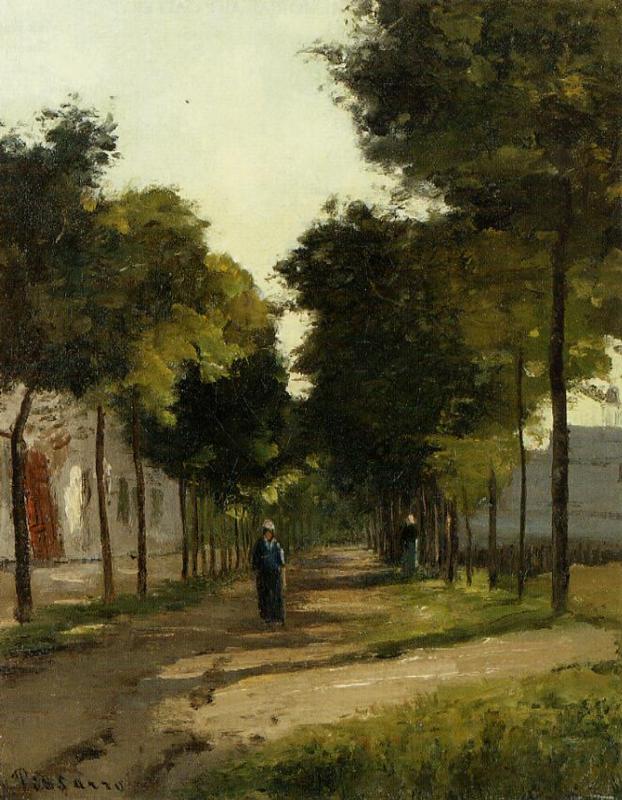The painting depicts an impressionist outdoor scene reminiscent of Monet, characterized by its impressionist style with blurry, small brush strokes coming together to form the image. This artwork, signed in the lower left corner by "Pissarro," features a footpath flanked by rows of tall, thin trees with fluffy, ball-like clusters of green and mossy yellow leaves. The path extends through the center of the image with a woman, in a long blue dress and white hat, appearing just left of center, suggesting depth and distance. Behind her and partly obscured in the shadows, there is a second figure, wearing a white hood, black top, and bluish-green skirt. On either side of the path, white or light gray buildings are partially visible, adding layers to the composition. Above the trees, the sky is rendered in shades of grayish-blue with hints of yellow. The setting evokes a serene daytime scene with vibrant colors, including hues of green, brown, gray, blue, and orange.